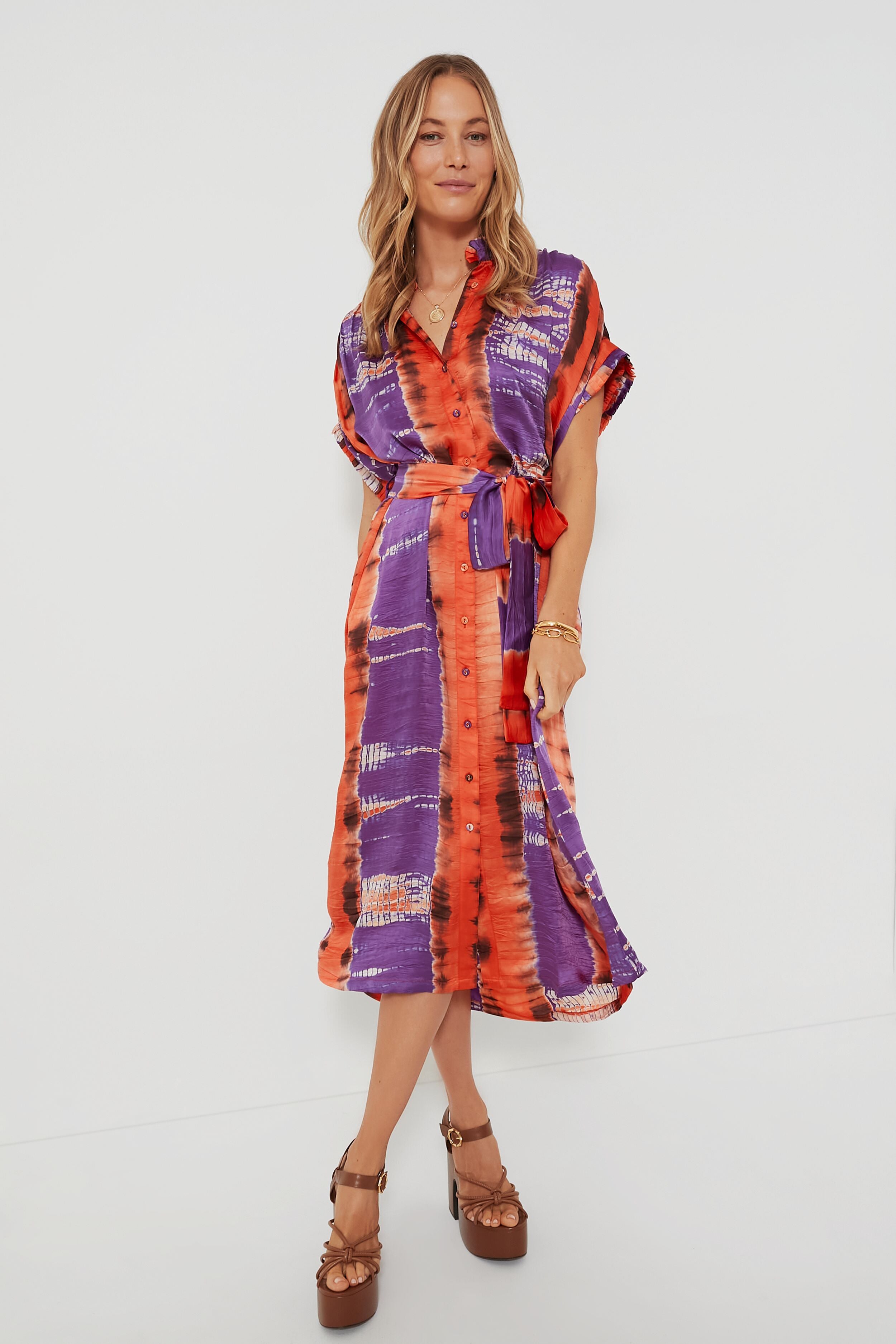In this fashion photograph, a woman with long, slightly wavy blonde hair stands against a plain white background, posing for the camera. She is a white female wearing a brightly colored, eye-catching dress that combines shades of purple, red, orange, and some black. The dress features a small ruffled collar, button-down front, and loose, rolled-up sleeves that stop just below the shoulder. It includes a self-belt made of the same material, cinching the waist. The dress falls to just below her knees and displays a tie-dyed batik pattern. Accessorizing her outfit, she wears a gold medallion necklace and several gold bracelets on her hands. Her right arm is slightly forward over her thigh, possibly holding the skirt of her dress, while her left arm is positioned in front of her. She completes her look with brown, strappy platform sandals, which have multiple straps over the toes and buckle around the ankle. The platform heels are several inches tall, showcasing her white nail polish.